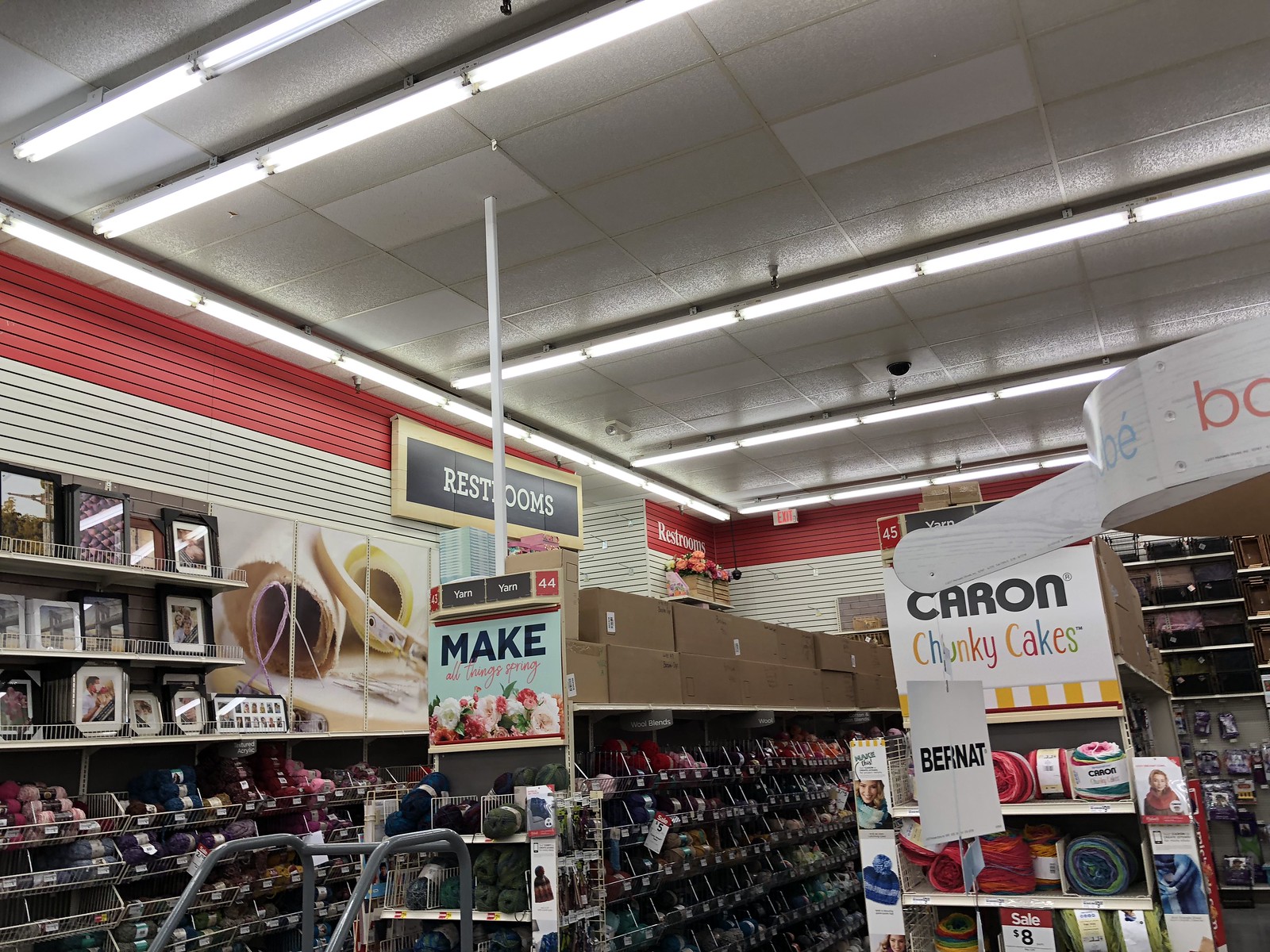This photograph, taken inside a likely Michaels craft store, captures a vibrant and detailed corner of the arts and crafts section. The store features white and red walls, a common design in Michaels stores, and is brightly lit with fluorescent lighting embedded in the paneled ceiling. The aisles are stocked primarily with rows of multi-colored yarn, prominently including "Caron Chunky Cakes" priced at eight dollars, and "Bernat" brand yarn. Three shelves on the upper sections of the aisles display various photo frames. Signs at the aisle end caps promote crafting, with one reading "Make All Things Spring" and another with an image of flowers simply saying "Make." In the far left corner of the image, there's a sign indicating the restrooms. The setting exudes an industrial, retail atmosphere with acoustic ceiling tiles and neatly organized crafting supplies, encouraging customers to embark on their creative projects.